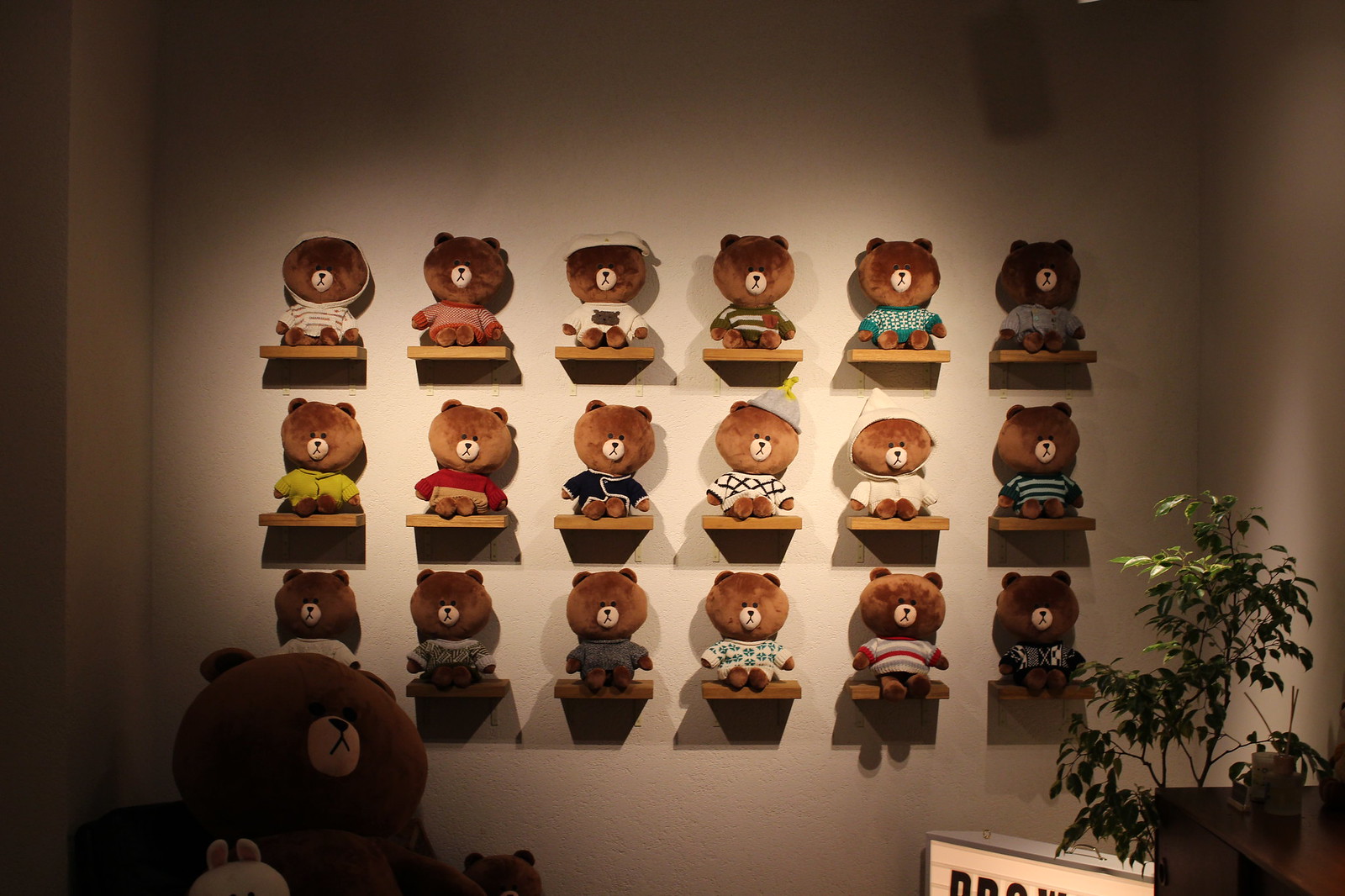The image showcases a display of 18 identical brown teddy bears, each with an enlarged head and a smaller body, arranged in a 6x3 grid on a cream-colored or tan wall. Each bear, characterized by its medium to dark brown fur, has a light tan nose with a brown embroidered mouth and nose. They sit on individual horizontal wooden shelves, dressed in unique outfits ranging from sweaters with stripes and front closures to hoodies, and some even donning little hats. The bears' various clothing styles add a whimsical charm to the uniformity of their large heads and small ears.

In the lower left corner of the image, a significantly larger version of these teddy bears sits on a dark-colored chair, accompanied by a smaller bear and a white rabbit, which has pink ears visible. In the lower right corner, a tree-like houseplant and a wooden shelf with several objects, possibly aroma diffusers, can be seen. Adjacent to this setup is a partially visible backlit sign with black lettering, standing on the floor. The background settings and elements, like pottery on a nearby table or credenza, add to the cozy and playful atmosphere of the display.